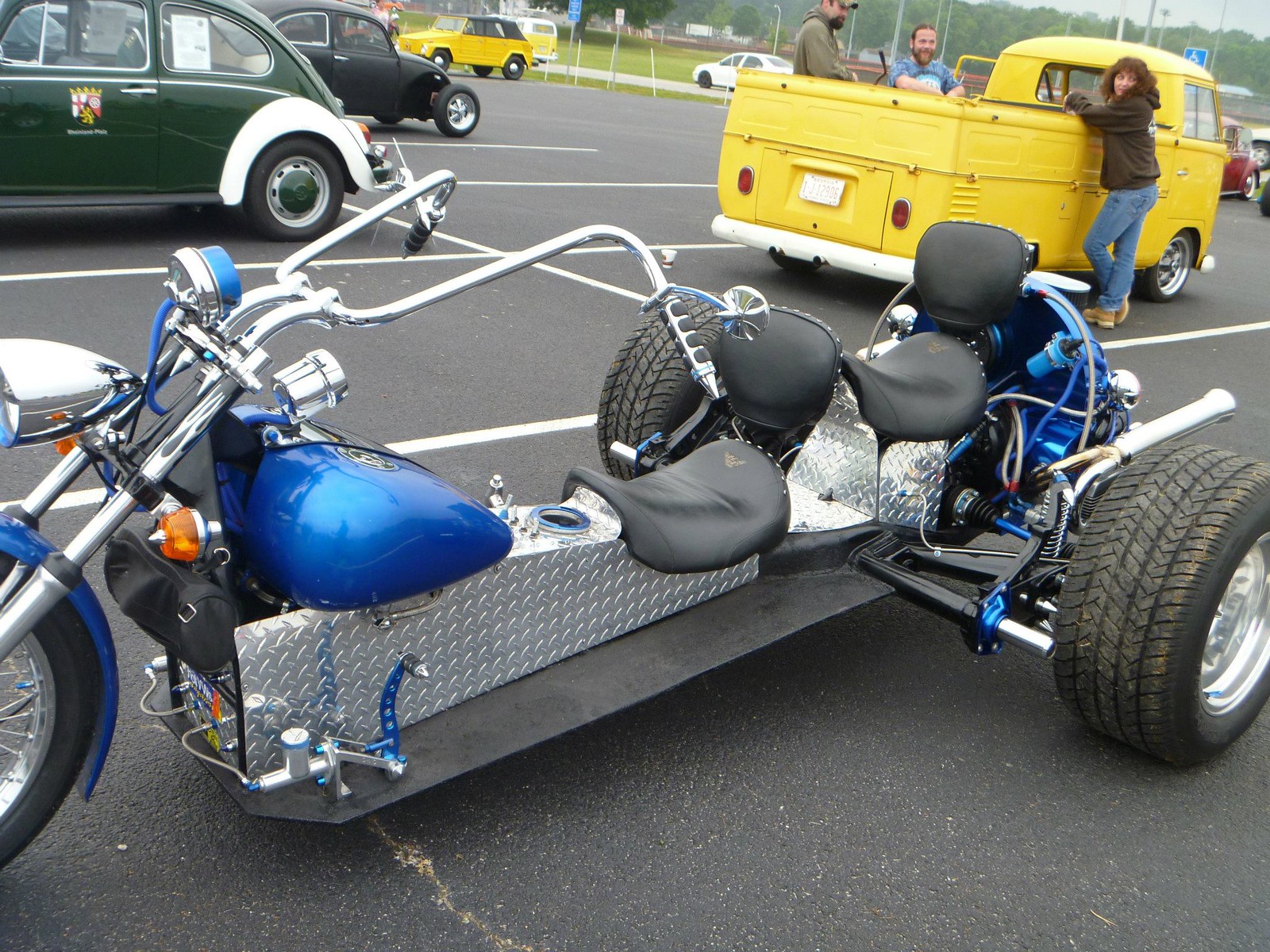This daytime photograph captures a lively parking lot scene filled with interesting vehicles and people. Dominating the foreground is an unusual, three-wheeled motorcycle, showcasing an extended build with long, low handlebars. The motorcycle features chrome accents, a blue tank and fender, large chrome handlebars, and a distinctive chrome headlight. Its seating arrangement is unique, with a formed leather seat at the front and a secondary black seat with a backrest towards the rear; large, wide tires with chrome rims complete its striking appearance. Notable is the blue element in the engine area behind the seats. 

In the upper left corner, a green VW Bug with a white bumper is parked next to a black VW Bug. Towards the far edge of the parking lot, a yellow car with a contrasting black top stands out, and adjacent to it is an old yellow pickup truck with a deeply rounded front and spacious back. Three people – one woman and two men – are gathered around the pickup truck, adding life to the scene. The background of the parking lot is dotted with more vehicles, patches of grass, and some trees, providing a picturesque setting for this eclectic collection of automobiles and onlookers.